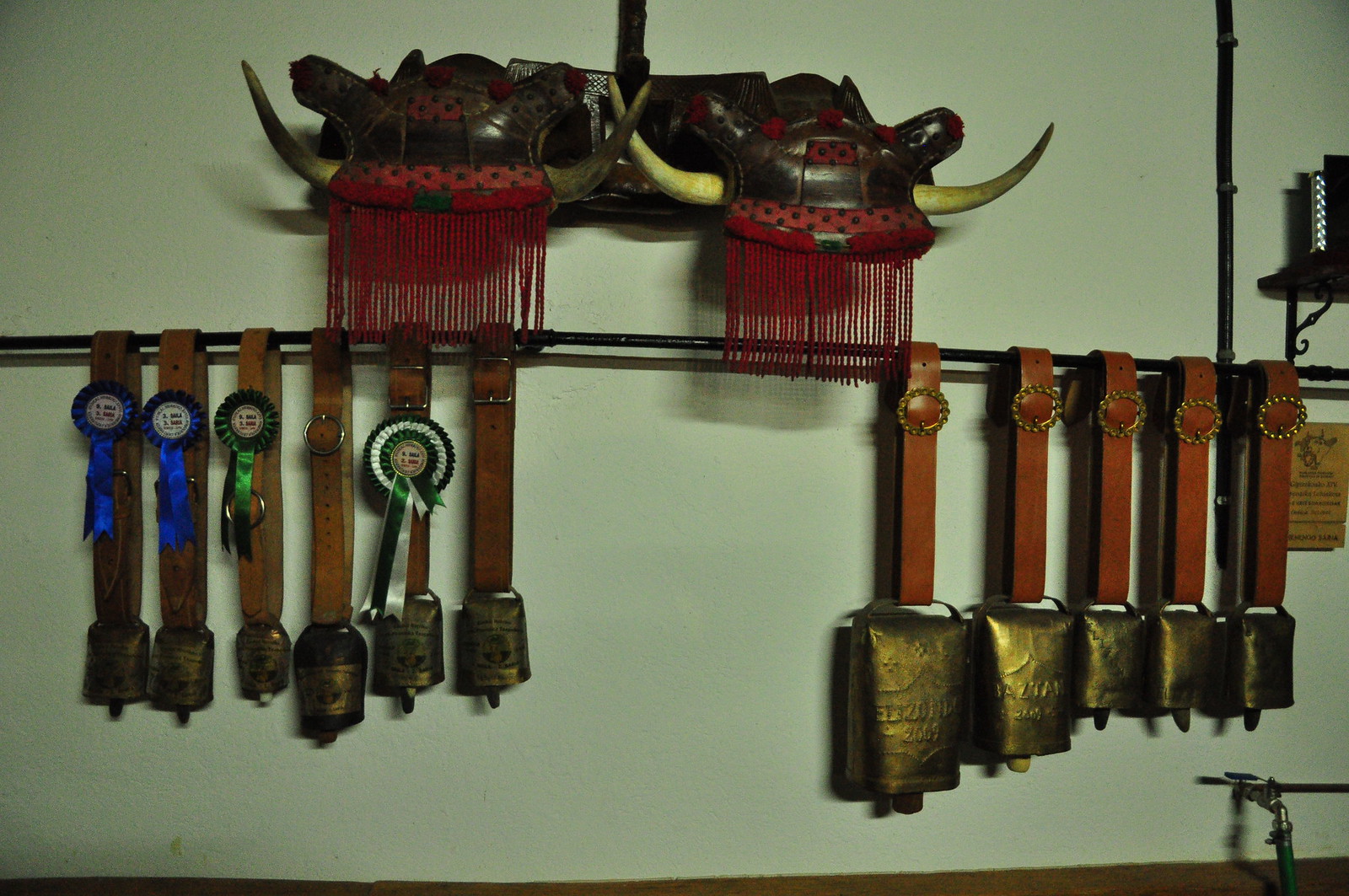This color photograph depicts a dense, indoor display of various cowbells and related memorabilia mounted on a grayish-white wall. A horizontal bar or thick wire spans the image, from which numerous brass cowbells hang, each secured by reddish-brown leather straps that feature decorative buckles. The metal of the cowbells displays a rich patina, suggesting they are antique. Several of these cowbells are adorned with prize ribbons—two blue ribbons, a green ribbon, and another ribbon striped in green, white, and red—possibly awards from county or state fairs. Above the cowbells, two Viking-style helmets with steer horns and dark red fringe are prominently featured, adding a historical or mythological flair to the display. Shadows cast by these items add depth to the photograph. In the top-right corner, there are additional shelves, though the contents remain indistinct. Overall, the scene is a detailed tableau of rustic charm and historical artifacts.